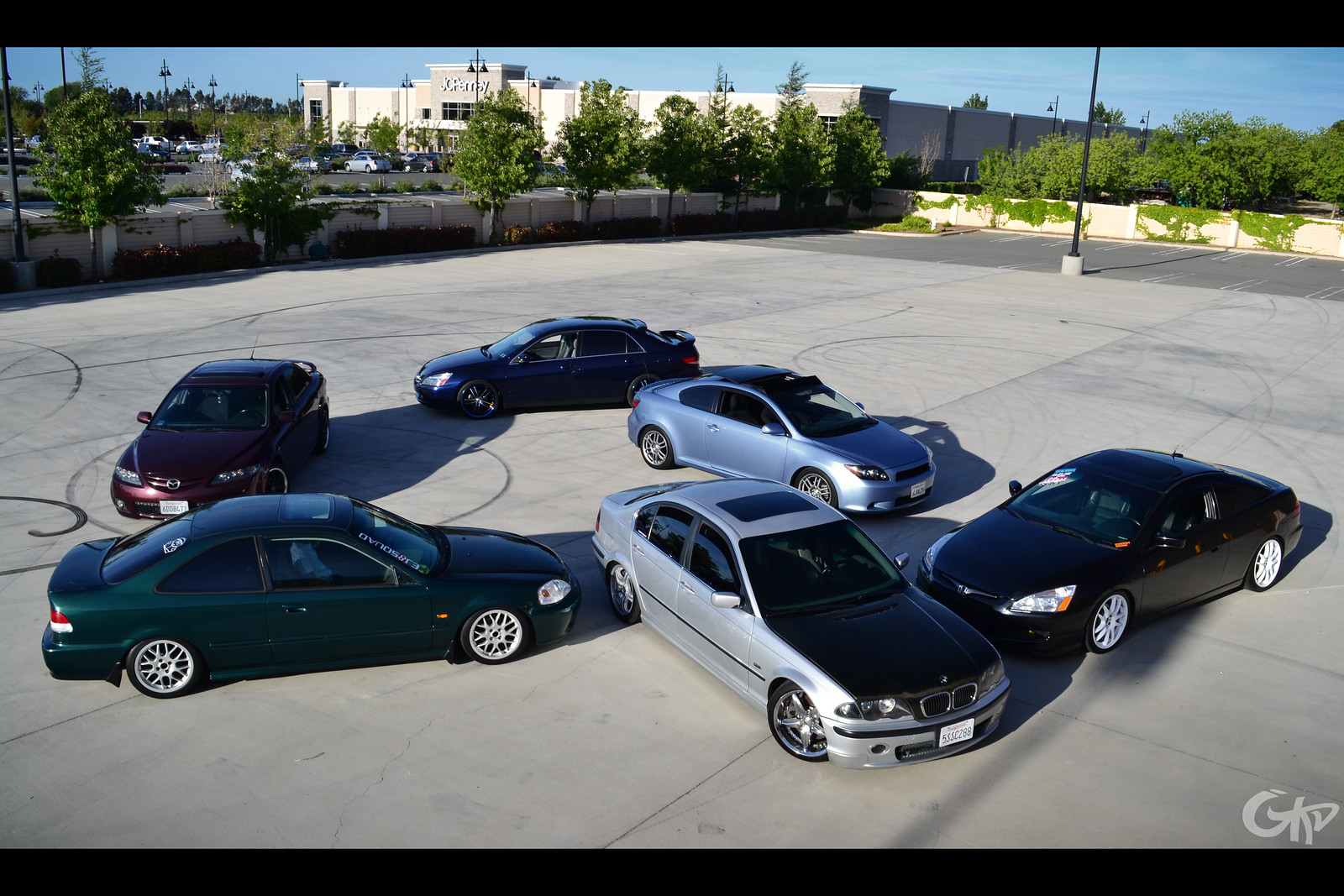In a busy American parking lot, six automobiles are arranged in a staggered circular formation, reminiscent of a staged artistic display. The surface bears the evident marks of tire spins, hinting at deliberate maneuvers likely executed for a visual effect. Behind this dynamic arrangement stands a J.C. Penney store, a light post, a fence, and a second parking area lined by trees. The variety among the vehicles is notable; while the specific brands mostly remain anonymous, a Honda and a BMW are clearly identifiable. The cars exhibit a range of colors, with four sporting darker shades like deep blue and black, and two covered in lighter hues such as silver and metallic blue. Judging by the style and position of the license plates, the scene appears to be set in the United States.